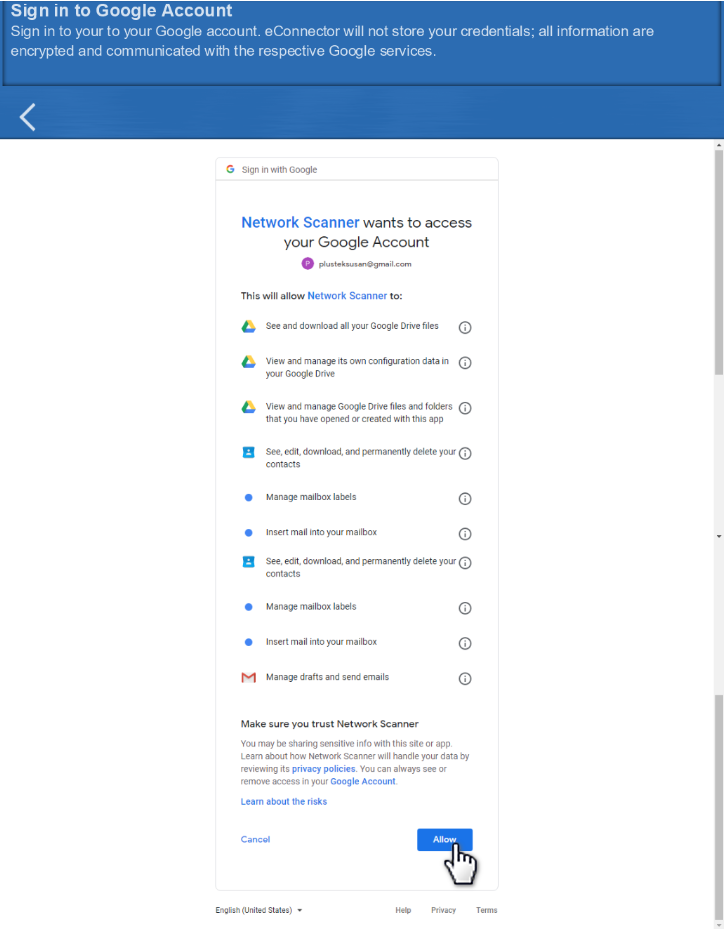This screenshot depicts a web page prompting the user to sign into their Google account. The page features a blue header at the top with the text "Sign in to your Google account." Below this header, a back arrow is situated on the left-hand side. 

Centered on the main part of the screen, there is a prominent "Sign in with Google" prompt. A message indicates that "Network Scanner" is requesting access to the user's Google account, specifying the user’s email address and detailing the permissions requested. These include viewing and downloading all Google Drive files, managing configuration data, accessing and managing Drive files created with the app, editing and deleting contacts, and managing mailbox labels, drafts, and emails.

The page cautions users to ensure they trust "Network Scanner" as sensitive information may be shared with this site or app. It also provides a link to learn more about "Network Scanner" and details on managing privacy policies. Users are reminded that they can always see or revoke access from their Google account.

At the bottom right of the screen, there is a prominent "Allow" button, indicated by a hand icon.